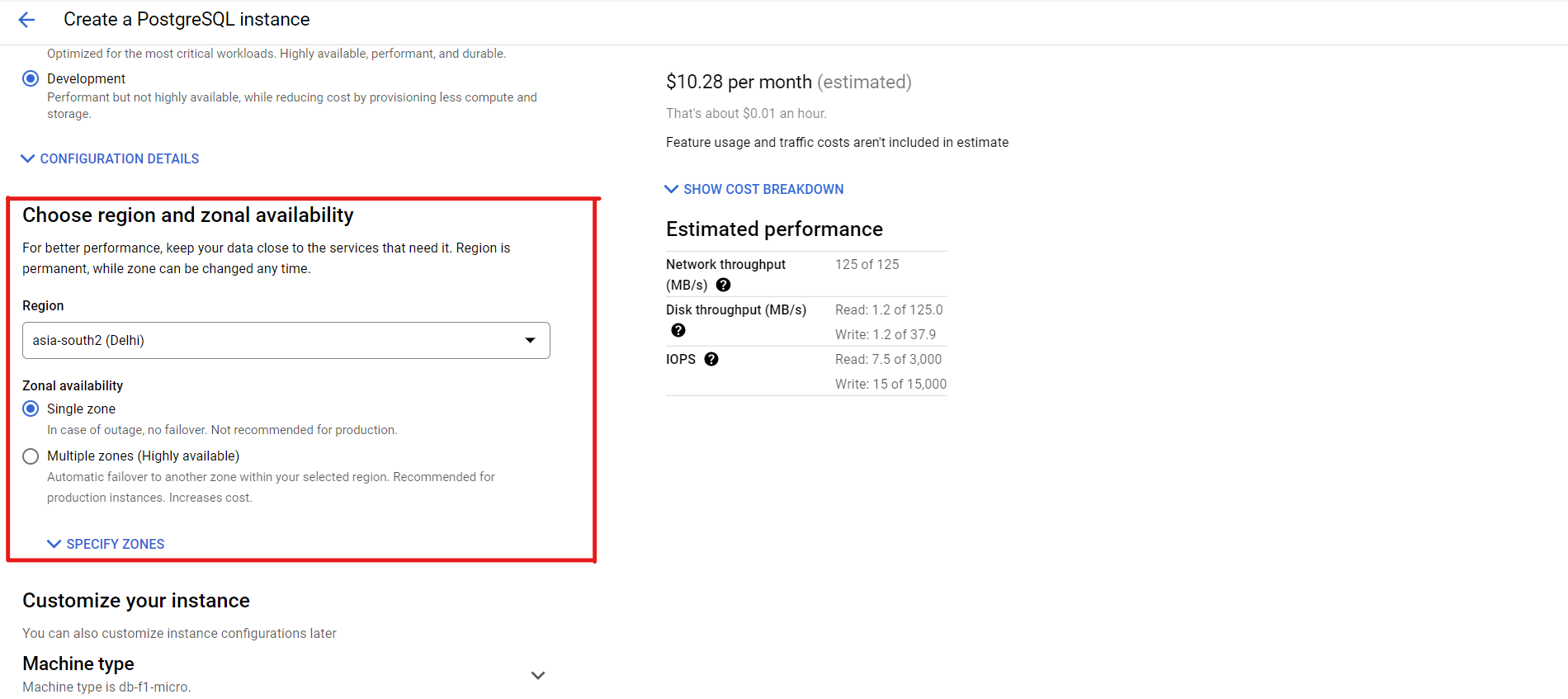This image displays a web page providing detailed information about creating a PostgreSQL instance. The text emphasizes optimization for the most critical workloads, highlighting attributes such as high availability, performance, and durability. Two options are presented: one optimized for development and performance but not highly available, focusing on cost reduction by allocating fewer compute and storage resources, costing an estimated $10.28 per month (approximately $0.01 per hour). The estimation excludes future usage and traffic costs. Additionally, the page provides an estimated performance breakdown, detailing network throughput, read and write speeds in megabytes per second (MB/s), and input/output operations per second (IOPS). The network throughput ranges from 1 to 5 MB/s. Read speeds are specified as 1.2 MB/s out of a potential 5.0 MB/s, while write speeds are 1.2 MB/s out of 7.9 MB/s. The IOPS metrics are 7.5 for reads out of 3,000 and 15 for writes out of 15,000.